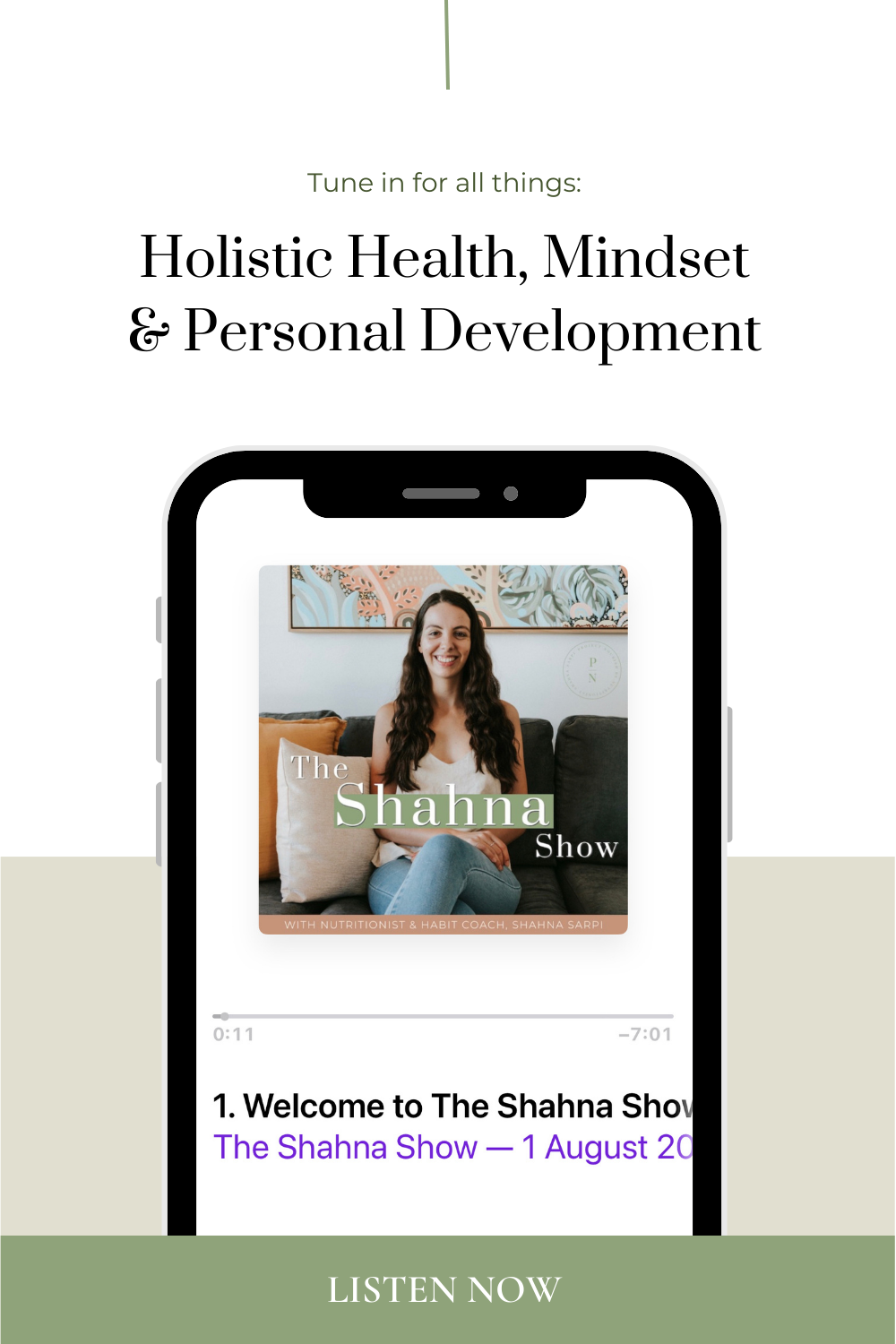The central focus of the image is a stylized eye, predominantly green at the top. Above the eye, there is a green text that reads, "Tune in for all things." Directly below this, black text continues with, "holistic health, mindset and personal development." The entire image features a white background.

At the bottom of the image, there is a picture of a smartphone displaying a video. The smartphone also has a white background. The video shows a woman sitting on a dark green couch adorned with orange and white cushions. The woman is dressed in blue jeans and a white vest. Behind her, a white wall features a brown picture frame. At the bottom center of the video, text reads, "The Shana Show," with "Shana" highlighted against a green background. Below this, more text states, "with Nutritionist and Herpes Coach Shana Sap," written in white against a light brown background. The video playback indicator shows that the video is at 0:11 seconds of a total 7:01 minutes.

Beneath the video, additional text includes "1. Welcome to The Shana Show," followed by "The Shana Show 1 August," written in purple. At the very bottom, a green button with the text "Listen Now" invites further engagement.